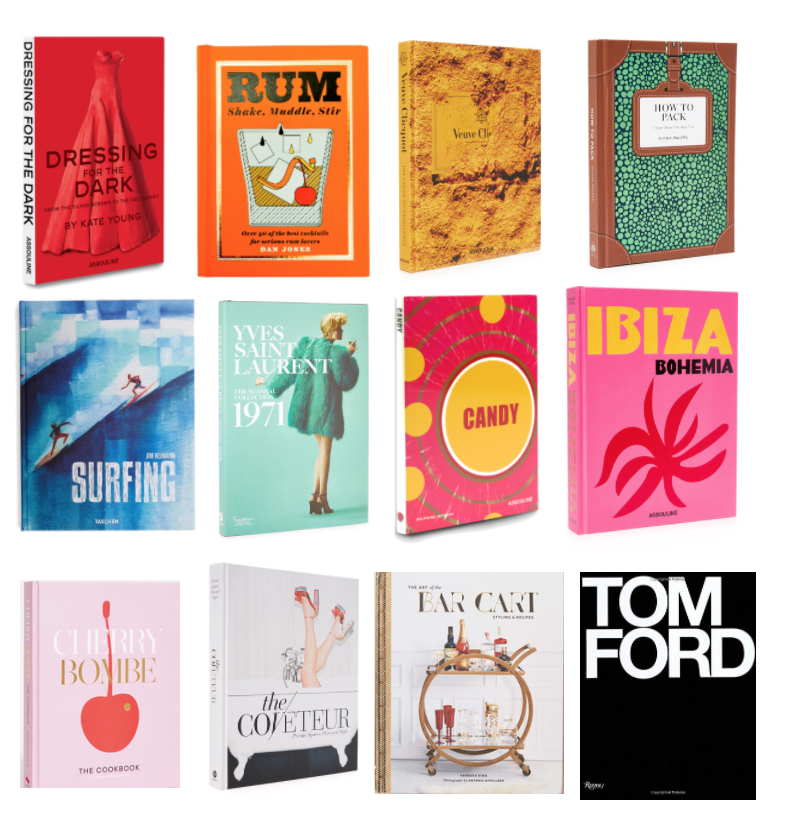This image showcases a meticulously arranged poster featuring the covers of twelve distinctive coffee table books against a pristine white background. The top row presents "Dressing for the Dark" with its angled display revealing a white spine and a vibrant red cover adorned with a wedding dress. Adjacent to it is "Rum Shaken Muddle Stir" in a bold orange shade. Flanked next is a visibly aged book with tiny black writing, followed by "How to Pack" featuring a suitcase motif, also angled. 

In the second row, a book on surfing catches the eye alongside an album dedicated to Yves Saint Laurent. "Ibiza Bohemia," richly colored, sits next to "Cherry Bomb," and "The Covetor" and "Farcart" close the line. The bottom right row features "Tom Ford" in a sleek, solid black design with prominent white lettering. 

In the center, another book titled "Candy" is vividly detailed, presenting a yellow central circle with red "Candy" lettering, surrounded by red and smaller yellow circles, echoing the playful motif of sweets. 

This display, visually reminiscent of high-end magazine spreads or publishing advertisements, encapsulates a collection that spans fashion, lifestyle, and travel wisdom in an elegant and cohesive presentation.